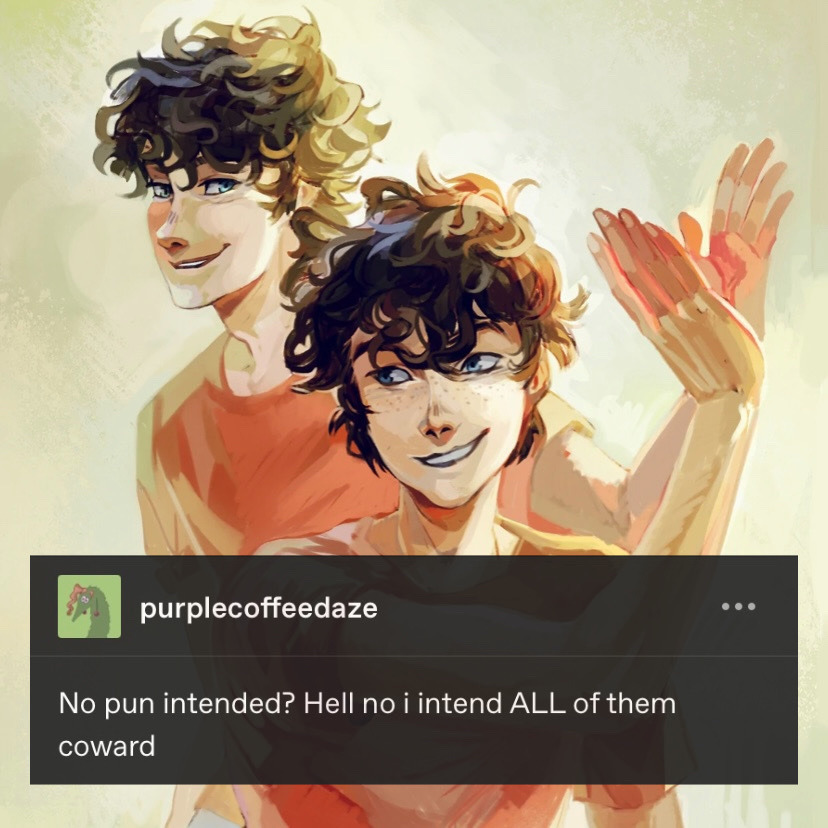The digital artwork features a central young boy with slightly curly black hair, blue eyes, and a sprinkling of freckles across his nose. He is donning a peach or orange-colored shirt. Behind him stands an older version of the same character, embodying the passage of time and growth. At the top of the image, a translucent bar displays the username "Purple Coffee Days." Beneath the username, a cheeky caption reads, "No pun intended. Hell no, I intend ALL of them, cowered," with emphasis on the word "ALL" through capitalization.